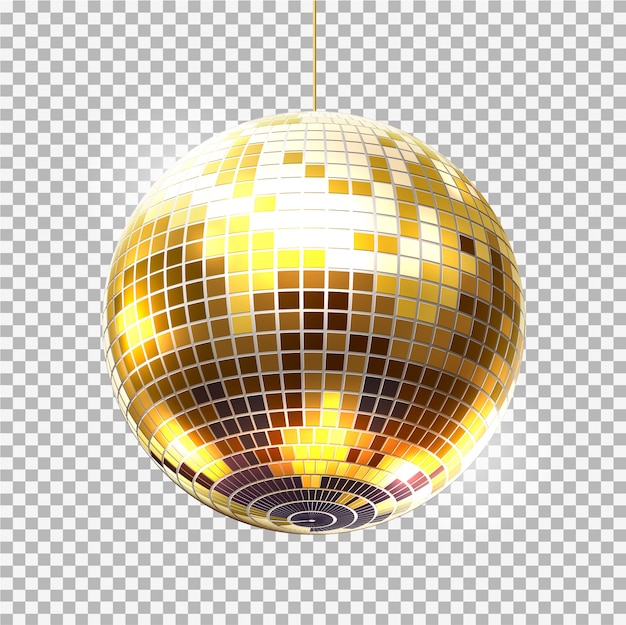The image is an illustration of a disco ball with a gold and white checkerboard pattern that creates a vibrant, shimmering effect as the tiles catch and reflect light. The disco ball is spherical, adorned with evenly sized square tiles, each of which exhibits a spectrum of colors from almost pure white to dark brownish-red, depending on their position relative to the light source. The upper left quadrant of the disco ball is particularly bright, indicating strong lighting, while the lower half is darker, enhancing the three-dimensional depth of the sphere.

The disco ball hangs from a thin wire that extends outside the frame of the image, suggesting it's suspended from a ceiling. The background features a small black and white checkerboard pattern that contrasts sharply with the glistening golden tiles of the disco ball. This background pattern covers the entire space not occupied by the disco ball, which is centrally positioned and takes up nearly half of the visual area. The perspective of the illustration appears to be slightly angled from below, emphasizing the ball's spherical nature and the dynamic play of light across its surface.